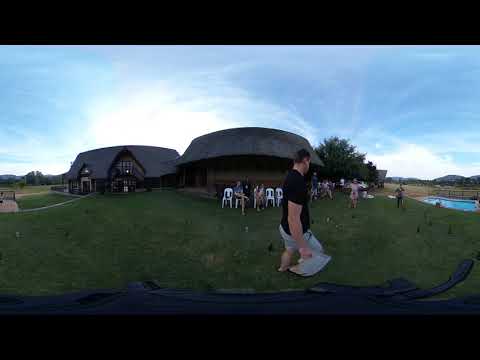In this vibrant park-like setting, the photograph captures a sunny day with a clear blue sky dotted with wispy clouds. Center-stage stands a man with short dark hair, dressed in a black short-sleeved shirt, gray shorts, and sandals, holding a piece of paper in his right hand. He's positioned on a lush green lawn. The scene is framed by two unique dome-shaped buildings in the background, each featuring double-dome structures and an alpine-style design with gray roofs and brown and white walls. Further behind this architectural focal point stretches a view of distant mountains and a tree with dark green foliage. To the right, a small swimming pool is visible, encircled by a fence. Scattered across the setting are people engaged in various activities; many are seated on white plastic chairs while others stroll around. A long driveway runs along the left side. There's a palpable sense of community and leisure, enhanced by the picturesque and serene environment.